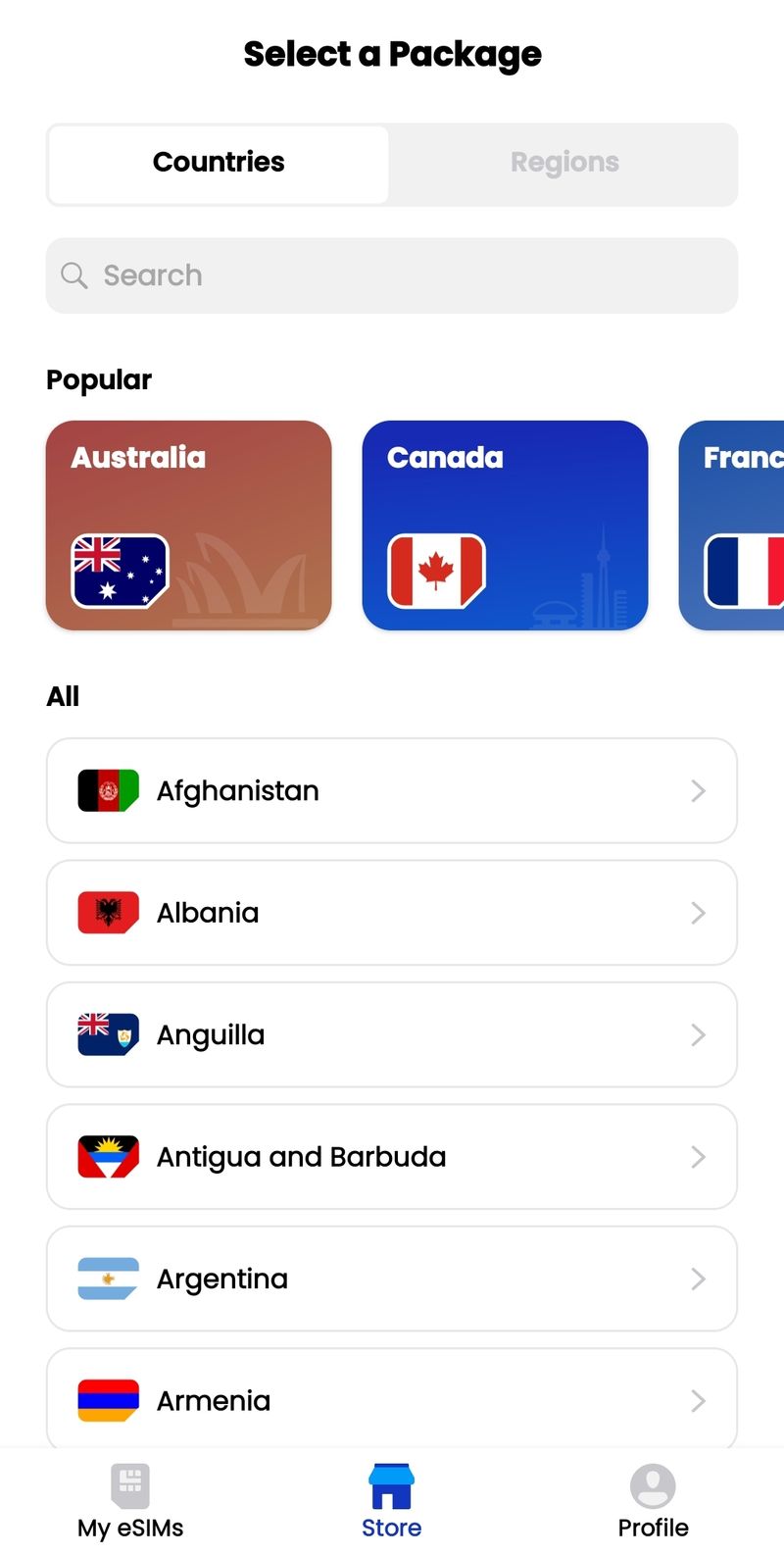The screenshot displays a user interface of an app designed to allow users to select various travel packages based on geographical distinctions. 

The layout features a clean white background with the title "Select a Package" prominently displayed in bold black text at the very top. Below this, users are presented with a toggle switch that allows them to choose between "Countries" and "Regions." The currently selected option, "Countries," is highlighted in white, while "Regions," unselected, is grayed out.

Beneath the toggle switch is a gray search bar for easy navigation and a smaller black text caption reading "Popular." This section features a horizontally sliding selection of country icons representing Australia, Canada, and France. Each icon displays a small flag in the bottom-left corner and the country's name in the top-left. The backgrounds of these icons are color-coded: rusty orange for Australia, dark blue for Canada, and light blue for France. The backgrounds also showcase famous architectural landmarks from each country, such as the Sydney Opera House for Australia.

Further down, another section labeled "All" in black text offers a grid layout of selectable white boxes, each containing a flag and corresponding country name. Countries listed here include Afghanistan, Albania, Angola, Antigua and Barbuda, Argentina, and Armenia.

At the very bottom of the interface, three icons provide navigation options: "My eSIMs," "Store," and "Profile." The "Store" icon is highlighted in blue, indicating the user's current location within the app, while the other two icons are grayed out.

This detailed layout provides an intuitive and visually organized method for users to explore and select travel packages based on specific countries.